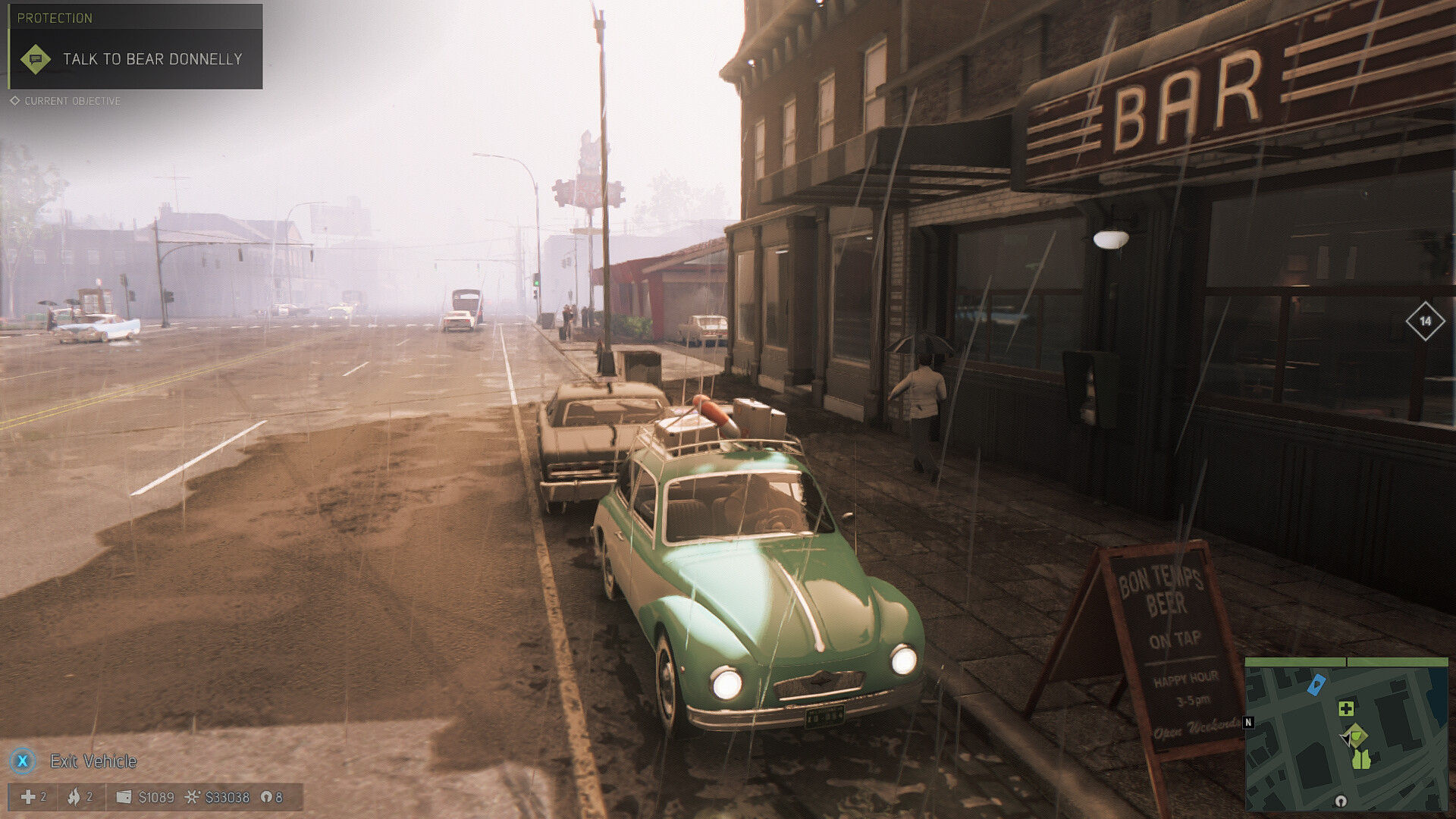This image captures a retro-themed scene from a video game, likely played on an Xbox, highlighting a sepia-toned street setting. The screen depicts a road lined with several vintage buildings on the right, including a prominent bar and other adjacent shops. One of the buildings has a visible placard advertising "beer on tap" along with its brand. The environment features a variety of older vehicles, including a distinctive green Volkswagen Beetle with luggage boxes tied to a roof rack. Additional cars in the scene include a grey one and a brown one positioned further back. The road itself appears dusty and grimy, adding to the overall antiquated feel of the scene. A bus and a white car can be seen in the background, further populating this nostalgic urban landscape. Additionally, a character is visible walking away in the mid-ground, contributing to the bustling atmosphere. The top left corner of the screen displays the objective "Talk to Bear Donnelly," providing context for the player's next action within the game.